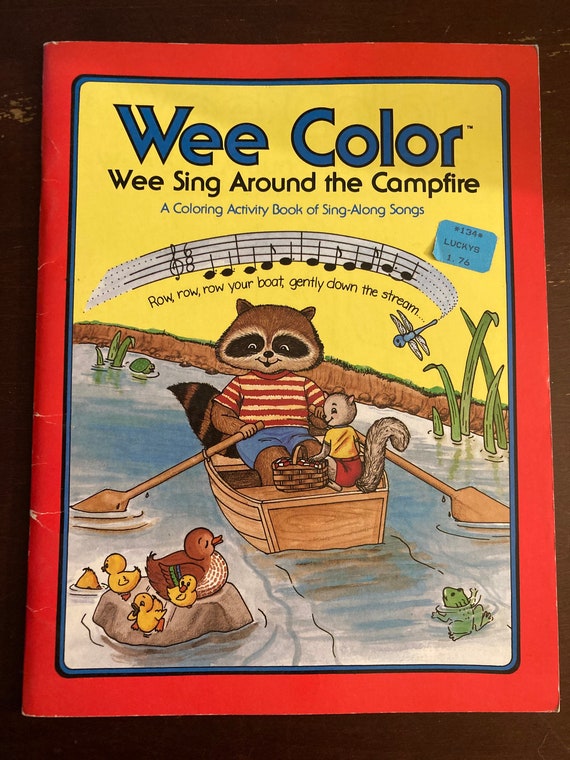This photograph captures the cover of an old-school children's coloring activity book from the 1970s or 1980s titled "We Color, We Sing Around the Campfire: A Coloring Activity Book of Sing-Along Songs." The cover features a whimsical illustration of a raccoon rowing a small boat with a squirrel holding a picnic basket, depicted in a simple cartoon style for kids. They are on a tiny river, with plants emerging from the water and a frog observing them. The animals are looking toward a mother duck and her four ducklings resting on a rock, with one duckling swimming. A dragonfly is also present in the scene. Below a line of musical notes, the cover specifies the song "Row, Row, Row Your Boat Gently Down the Stream." The book has a distinctive red border with a yellow middle section and is priced at $1.76, as indicated by a sticker, possibly purchased from Lucky's. The book itself is set on a brown, older wooden bench, adding to the nostalgic feel of the image.